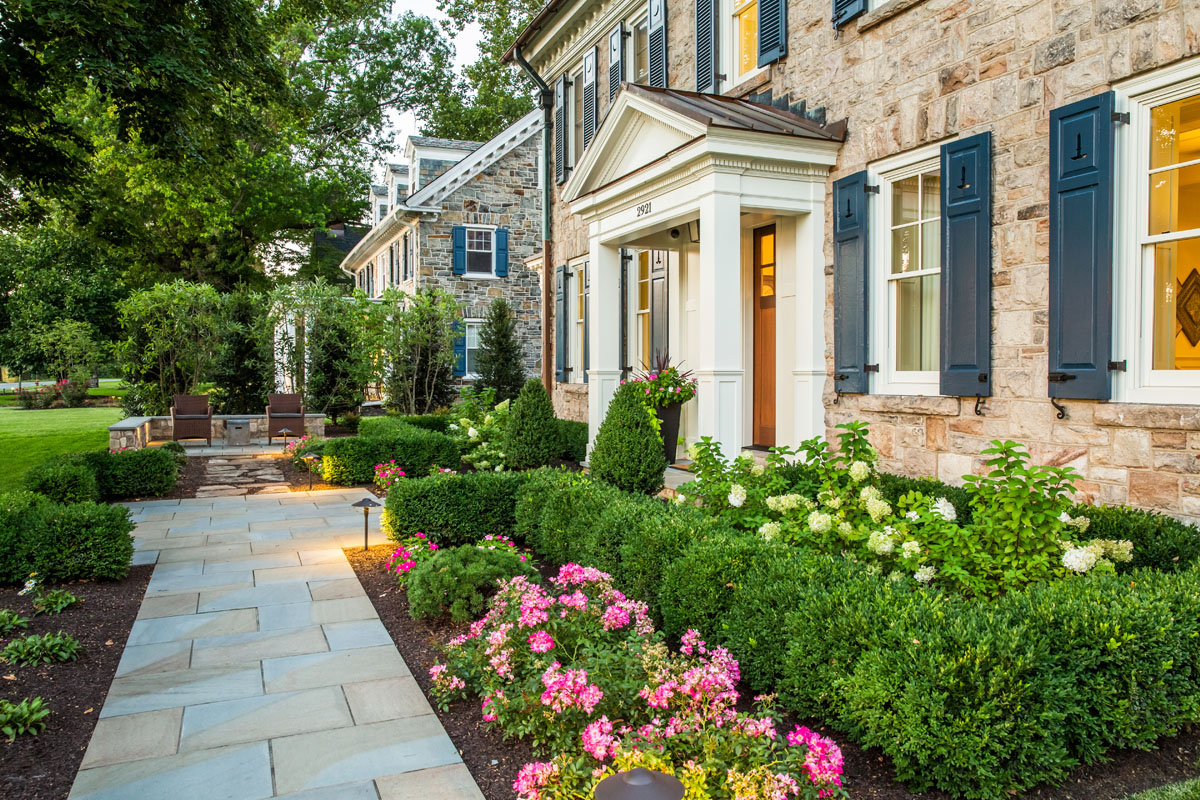The photograph captures the front view of a large, well-maintained brick house in a suburban neighborhood, presented at an angle as if standing at the end of the stone walkway leading to the front door. The house features numerous white-framed windows, each adorned with slate blue shutters that have cut-out candlesticks at their tops. Over the dark brown wooden front door is a pointed overhang supported by white columns, with the house number "2921" displayed above in black. The front yard is meticulously landscaped, showcasing vibrant green trimmed bushes shaped into flat rectangles, interspersed with pink flowers and white hydrangeas closer to the house. In the background, the similarly brick-built neighbor's house with matching windows and shutters is visible. The stone pathway, composed of tan and white paver bricks, bifurcates to each door and leads past two wooden chairs placed on the far left side, adding a cozy touch to the scene.